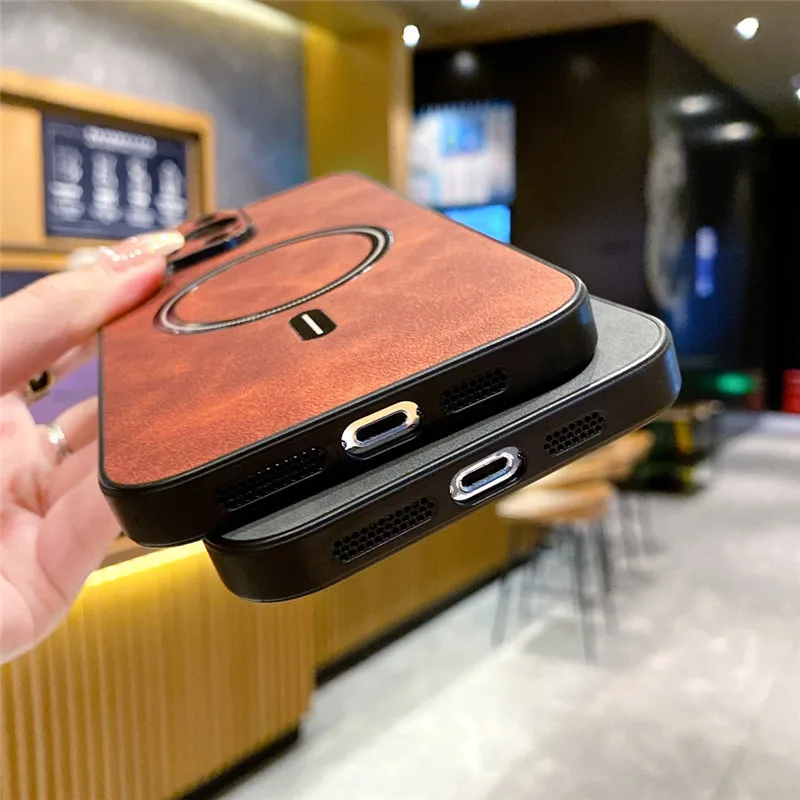This close-up photograph prominently features a woman's hand, with long, polished fingernails, holding two iPhones stacked one on top of the other. The upper iPhone sports a brown, leather-like case with a circle in the center, while the lower iPhone has a gray back barely visible due to the top phone covering most of it. The bottom phone’s chrome-edged charging ports and the black rubber rim of its case are noticeable. The background, though blurred, suggests a bar or café setting. The floor consists of large gray tiles, leading up to a counter with a yellow mustard trim. Behind the counter, black-legged stools with wooden seats are visible. The scene includes ambiguously detailed elements like additional seating and possibly television monitors on the gray walls. The overall focus remains on the two phones, with the surrounding environment providing context.